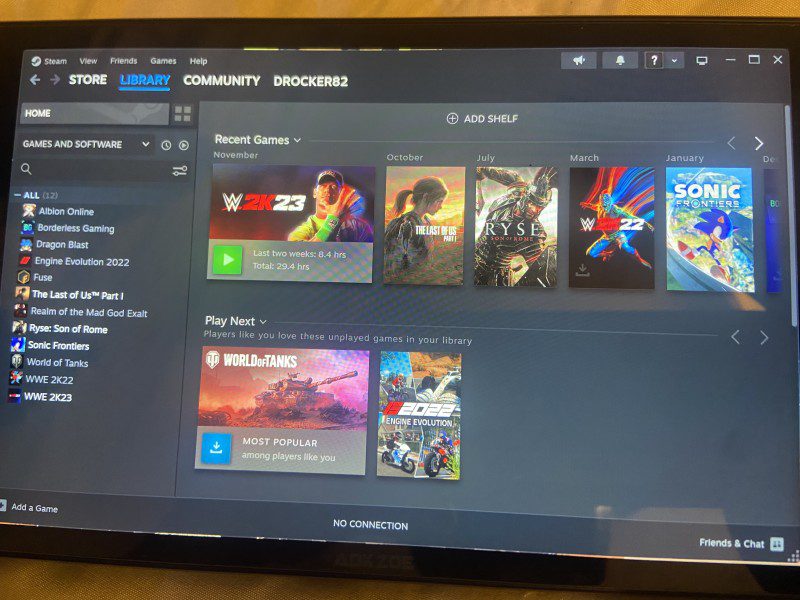This image showcases the Steam interface on a computer screen. The classic Steam logo is visible in the upper left-hand corner. Just below the logo, the main navigation options—View, Friends, Games, and Help—are listed. Under these options, there is a back and forward button for easy navigation, followed by buttons for the Store, Library (which is currently selected and highlighted in blue with an underline), Community, and the user's profile name, DRocker82.

Just below the top navigation bar, there is a section listing games such as W2K23, The Last of Us Part 1, Ryse: Son of Rome, W2K22, Sonic Frontiers, and World of Tanks. It also highlights popular games among similar players, featuring 2022's Engine Evolution.

On the left side of the interface, a vertical list of the user's owned games is shown, including titles like I'll Be On Online, Borderless Gaming, Dragon's Blast, among others.

In the upper right-hand corner, there are the typical window control buttons (close, maximize, and minimize). To the bottom right, there is a section dedicated to Friends and Chat. The bottom bar in the middle indicates a "No Connection" status, and in the bottom left corner, there is an "Add a Game" button.

Overall, the interface provides a comprehensive overview of the user's game library, navigation options, and community interactions.